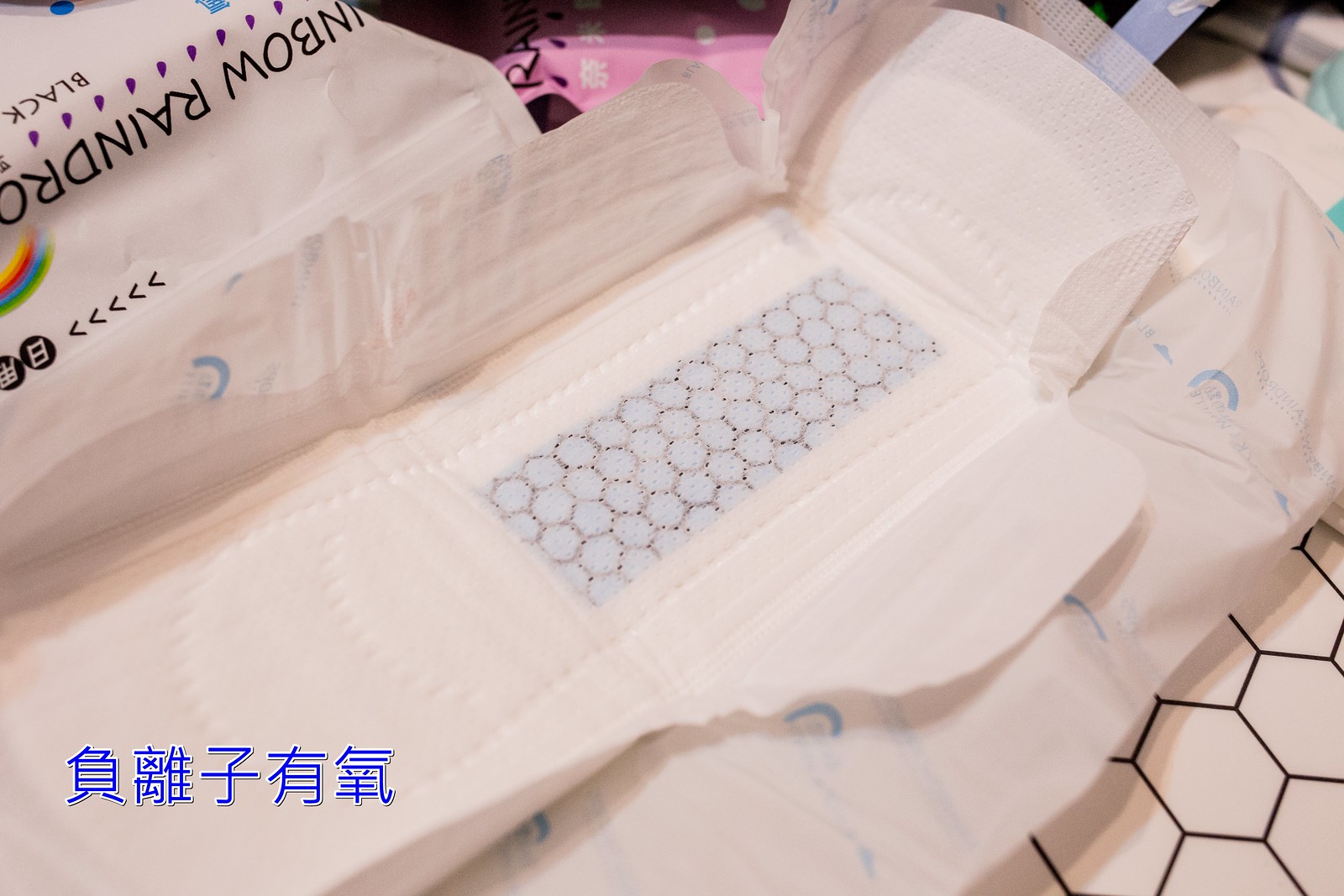The image captures a white sanitary pad for females, featuring wing flaps and a self-adhesive strip, unfolded to reveal its full shape. It is set against a white tile counter with a distinct beehive tile design. In the lower left-hand corner of the image, there is blue text that appears to be in Japanese or another Asian script. To the side, a partially visible package, which originally contained the sanitary pad, is present. The package is predominantly white with a rainbow graphic in green, blue, red, and yellow and contains black lettering, including the words "rainbow" (which is upside down). Despite a slight confusion with associating the item with diapers or tampons, it is clearly identified as a sanitary pad used for absorbing menstrual flow.